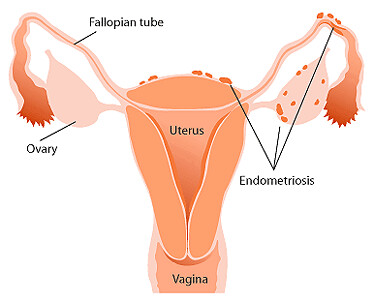This medical diagram illustrates the female reproductive system in detailed, light and medium pink hues, accented with dark orange on parts of the fallopian tubes. The central elements include the uterus, fallopian tubes, and ovaries, each clearly labeled with black, sans-serif font text. Though the text appears somewhat small, arrows efficiently direct the viewer's attention from these labels to their corresponding anatomical parts. The illustration prominently addresses endometriosis, indicated by brown dots dispersed on the ovaries, fallopian tubes, and the upper section of the uterus. The diagram is set against a white background with subtle gradient shading, enhancing the visual depth of this flat color illustration.